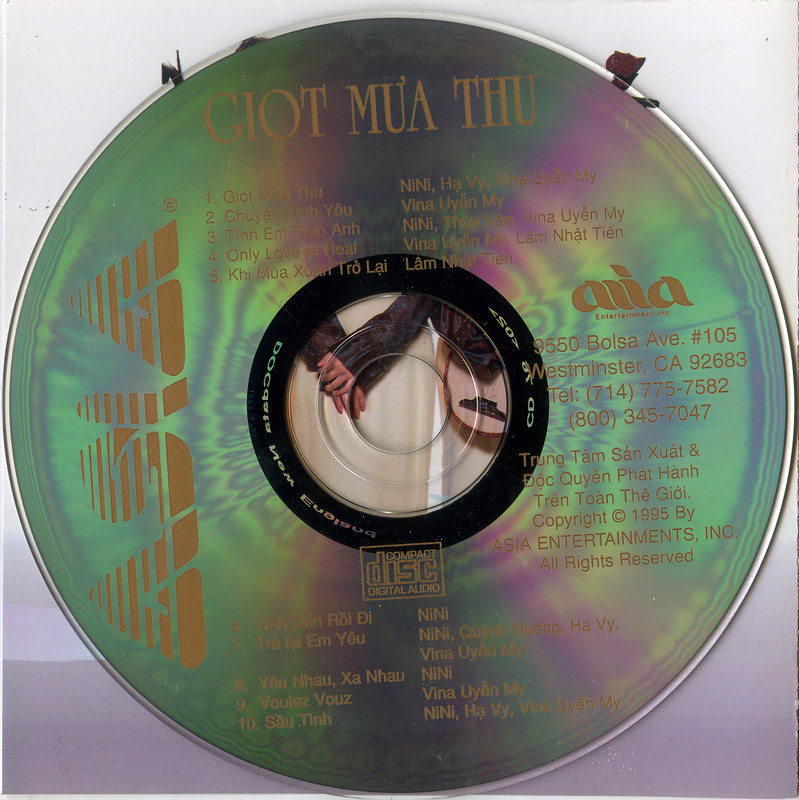The image depicts a CD titled "G I O T M U A T H U" by Asia Entertainment Inc., produced in 1995. The CD, devoid of a case, is resting on a piece of paper, partially covering an illustration of two women clasping hands. The disc itself has a clear surface with a tan or gold font and exhibits a reflective, rainbow-like sheen. It lists ten tracks, with the first five at the top and the remaining five at the bottom. The titles are mostly in Vietnamese, with one track, "Only Love is Real," in English. The right side of the CD displays the address "9550 Bolsa Avenue, Suite 105, Westminster, California, 92683," along with telephone numbers 714-775-7582 and 800-345-7047. The text also includes "Trung Tam San Suat" and "Doc Tuyen Phat Han," denoting its production details. The CD's copyright by Asia Entertainment is prominently noted.